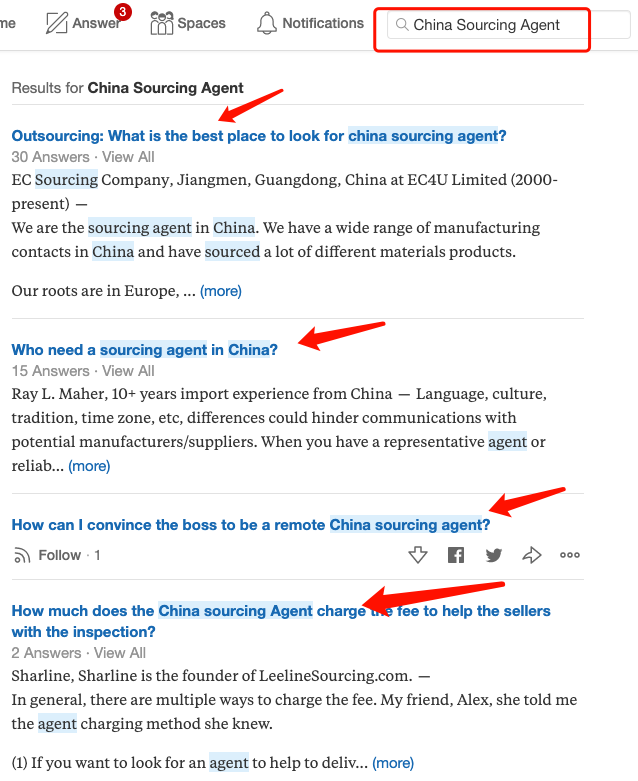Screenshot of search results for "China sourcing agent." The highlighted search box is prominently displayed at the top right corner of the screen. Several small red arrows point to different search results. The visible results include:

1. "Outsourcing: What is the best place to look for a China sourcing agent?"
2. "Who needs a sourcing agent in China?"
3. "How can I convince the boss to be a remote China sourcing agent?"
4. "How much does a China sourcing agent charge?" (This result appears to discuss the fees for helping sellers with inspections.)

Each result listed seems to have a corresponding answer.